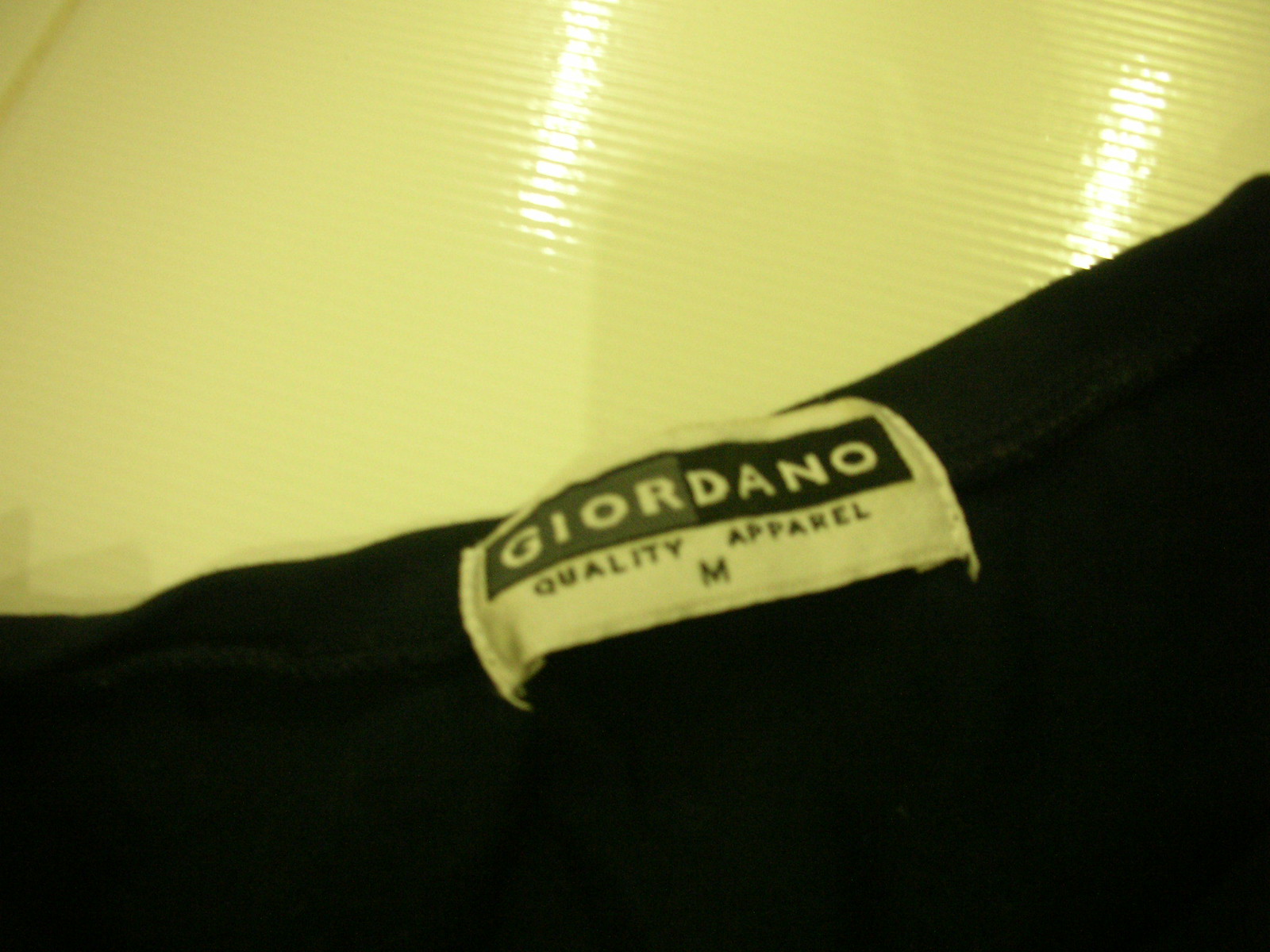A close-up image showcases a black garment displayed against a bright yellow, textured background. The backdrop, which appears shiny with light reflections in two spots, is likely a plastic material, distinguishing itself from the apparel. The garment is placed at an angle, with the narrower part positioned toward the lower left and the broader section extending to the upper right. The main focus of the image is the clothing tag, prominently featuring “Giordano” in yellow uppercase lettering on a black banner. Below, the tag reads "QUALITY APPAREL" in black uppercase letters and indicates the size "M" for medium.